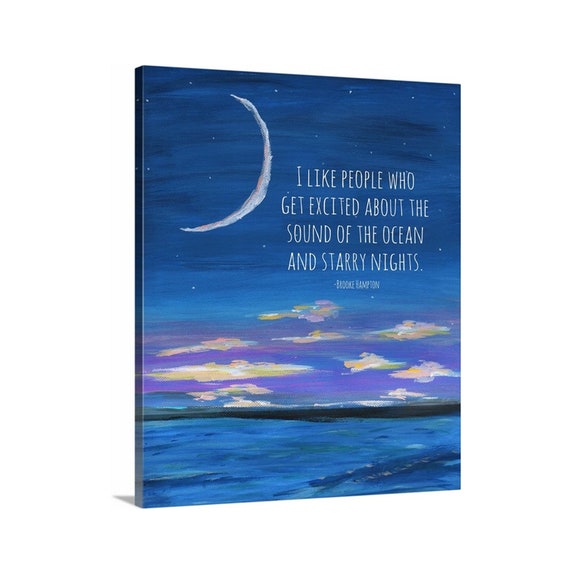This is a detailed, frameless painting that captures a tranquil night scene. In the top right corner, there's a quote that reads, "I like people who get excited about the sound of the ocean and starry nights," attributed to Brooke Hampton. The artwork predominantly features a dark blue sky adorned with a scattering of stars and a bright crescent moon positioned on the upper left. Beneath the quote, fluffy clouds in hues of white, yellow, orange, and pink suggest the gentle glow of sunset or sunrise against a subtly purplish backdrop. Below the clouds, a dark green horizon appears to transition into a mountainous silhouette, further enriched with layers of black to depict land. The bottom portion of the painting illustrates an ocean scene, textured with various shades of blue and green and accented by dark spots indicating waves, enhancing the natural beauty and serenity of the ocean at dusk.